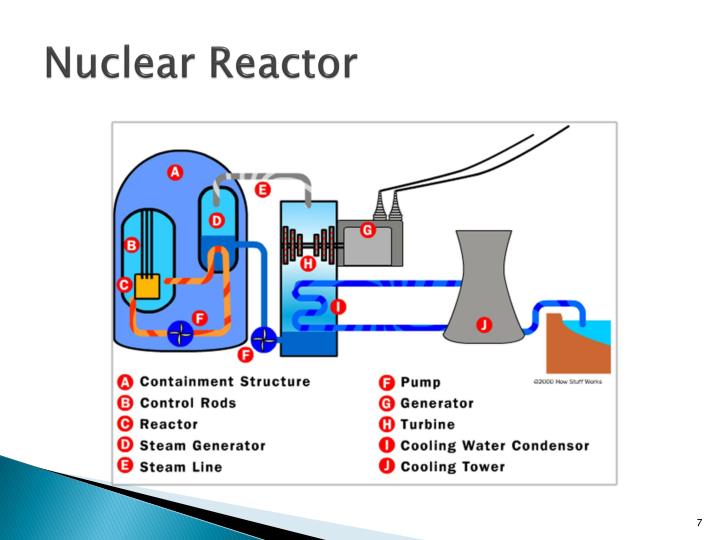The PowerPoint image displays a detailed model of a nuclear reactor. At the top, the words "Nuclear Reactor" are prominently written in black. The central area features a comprehensive diagram of the reactor, meticulously labeled with letters A through J, each corresponding to a distinct component. This labeling system includes a containment structure (A), control rods (B), reactor (C), steam generator (D), steam line (E), pump (F), generator (G), turbine (H), cooling water condenser (I), and cooling tower (J). The diagram effectively illustrates the flow of cooling water from the cooling tower (J) towards another water structure. The visual includes icons or shapes for each component, like the blue cylindrical containment structure and specific pathways for steam and water, making it a thorough and educational representation of the inner workings of a nuclear reactor.